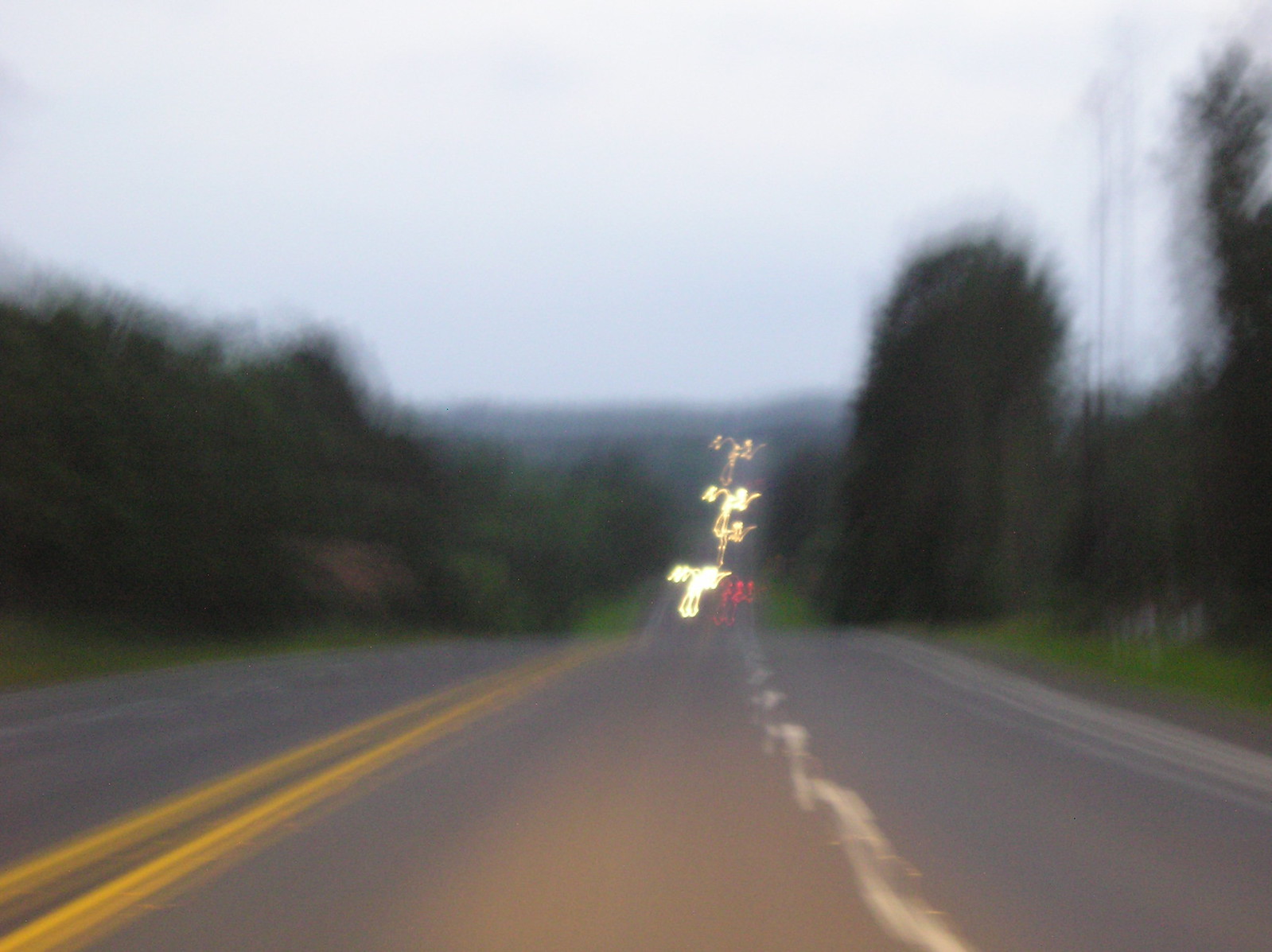This image depicts a blurry photograph taken on a highway. In the foreground, the road is visible with two lanes separated by a dotted white line. To the left of these lanes are two solid yellow lines which divide the opposing directions of traffic. Further left, another dotted white line can be seen. In the distance, a multitude of cars on the horizon emit a yellowish hue from their headlights, suggesting they are moving toward the photographer. The image captures the essence of a bustling highway scene, albeit with a lack of clarity due to the blur.